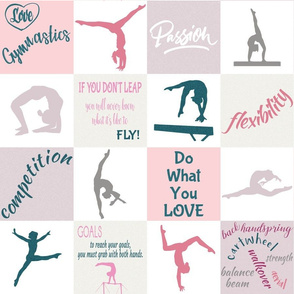This image is an art print featuring a collection of 16 squares, each showcasing various aspects of gymnastics. Half of the squares display vibrant figures of girls performing different gymnastics poses such as jumps, flips, cartwheels, back handsprings, aerial moves, and balanced stances on beams. The other half are adorned with motivational sayings like "Love Gymnastics," "Passion," "Flexibility," "Do What You Love," "If You Don't Leap, You Will Never Know What It's Like to Fly," and "To Reach Your Goal, You Must Grab With Both Hands." The overall color palette is a delicate mix of pink, purple, teal, and white, evoking a pastel theme. This artwork captures the essence of gymnastics and could easily be imagined as designs on shirts for young gymnasts, emphasizing the dedication and joy inherent in the sport.